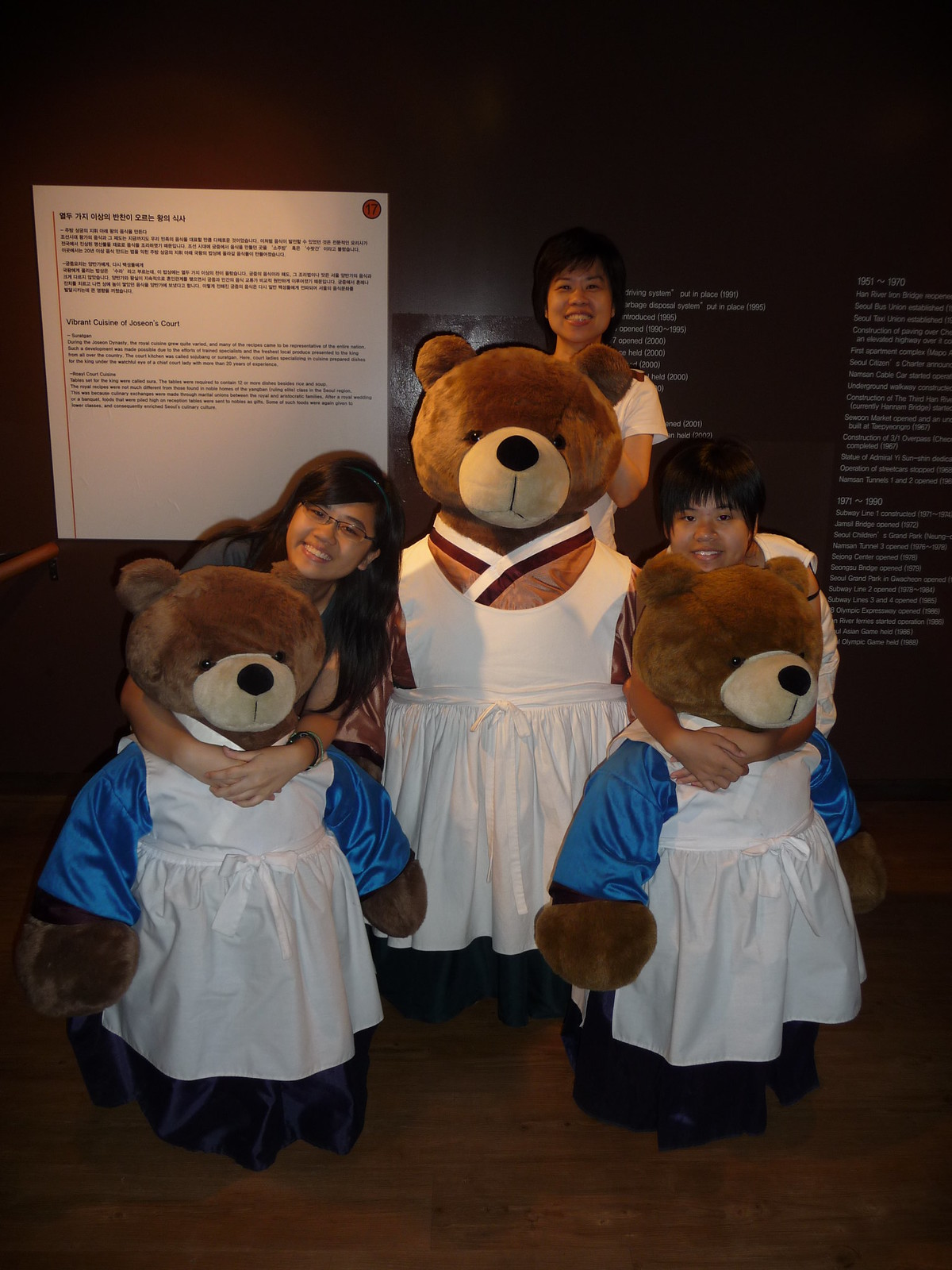This portrait-style photograph captures a charming group scene featuring three Asian girls and three large, life-sized teddy bears. The backdrop is a rich maroon wall adorned with a white poster board and a gray poster board, both featuring Asian writing. The floor is made of dark wood, adding a warm contrast.

The central figure is an older girl who stands behind a tall, plush teddy bear. This bear, almost reaching her neck, is dressed in a white dress with cut sleeves, giving it a distinct appearance. Flanking her are two younger girls, each hugging a smaller teddy bear from behind. These smaller bears are notably dressed in vibrant blue-sleeved dresses that extend just past the white fabric.

The teddy bears all share common features: brown faces, tan snouts, black, round noses, black eyes, and round, curly ears. Despite their height, the bears' feet are not visible in the photo. The two girls in front vary slightly in their appearance; the girl on the left has long black hair reaching her arms, while the girl on the right, with hair just to her ears, matches the hairstyle of the older girl.

The harmonious combination of elements—the maroon wall, the warm wooden floor, the vibrantly dressed teddy bears, and the affectionate poses of the girls—all contribute to the photograph's inviting and whimsical atmosphere.